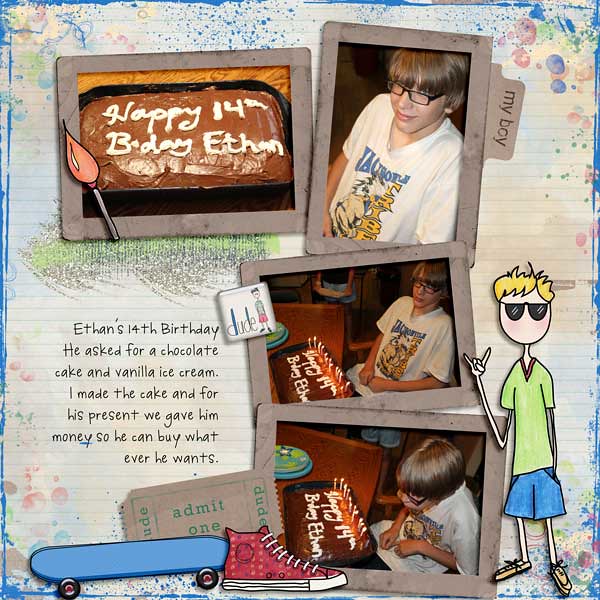The image is a montage celebrating Ethan's 14th birthday, possibly posted on social media. Central to the image is a homemade rectangular birthday cake with chocolate frosting, adorned with the message "Happy 14th Birthday Ethan" written in white, rustic-looking icing. Surrounding the cake are several photographs: one features Ethan, a young boy with dark-framed glasses, labeled "My Boy;" another shows him sitting in front of the cake, and the final image captures him blowing out 14 candles on the cake. Additional details include a blue skateboard, a red sneaker, a ticket reading "Admit One," and grungy paint splatters in the background. Text across the image notes, "Ethan's 14th birthday. He asked for a chocolate cake and vanilla ice cream. I made the cake, and for his present, we gave him money so he can buy whatever he wants."